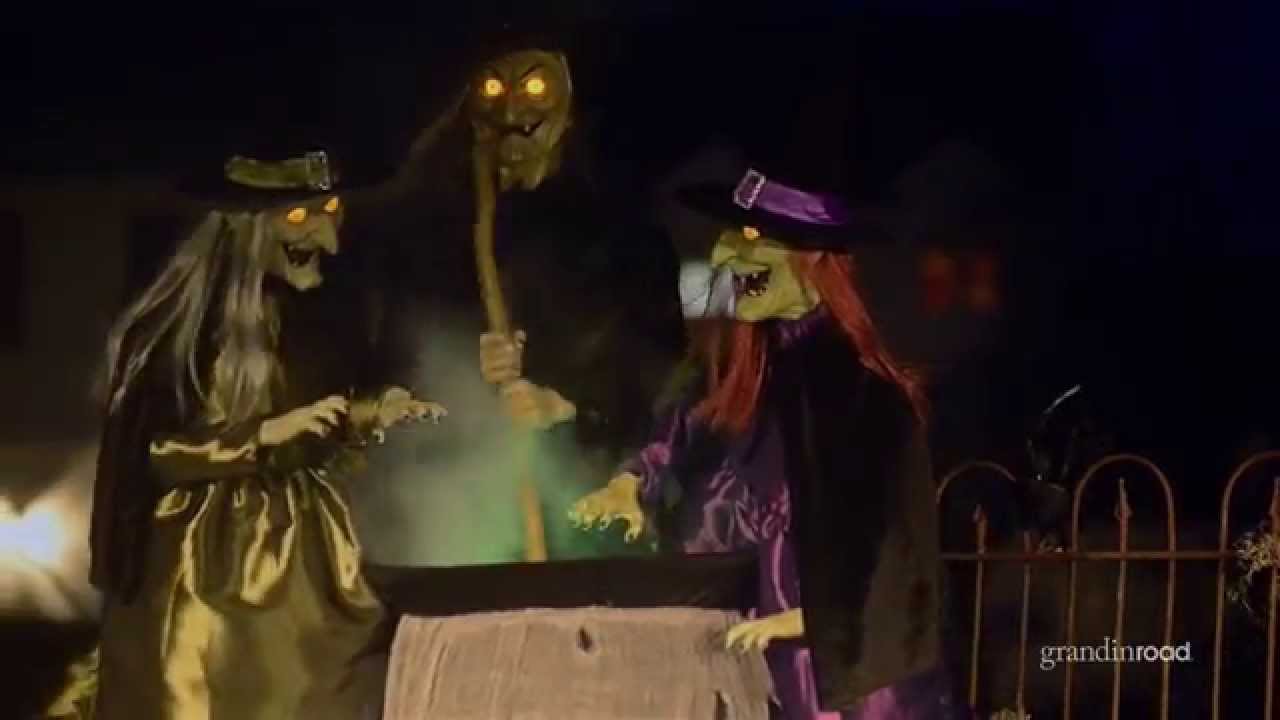In a captivating and spooky Halloween scene, three animatronic witches are gathered around a glowing, steaming cauldron that emits eerie green smoke. These witch decorations, designed with intricate details, showcase quintessential witchy traits. The witch on the left is clad in a gold dress and a black hat, her long gray hair flowing as she smiles sinisterly at the bubbling cauldron. The witch in the middle commands attention with her intense yellow glowing eyes as she looks directly at the viewer, stirring the cauldron with a long stick; her outfit shrouded in shadows yet emanating an air of malevolence. The witch on the right, dressed in a purple robe with a coordinating black cape and hat adorned with a purple ribbon, stands next to the cauldron looking to her right, her long red hair cascading down. A subtle hint of a fence on the right side suggests this scene could serve as an outdoor yard decoration. Notably, the bottom right corner of the image features the text “Grandin Road,” indicating the possible manufacturer of this Halloween display.